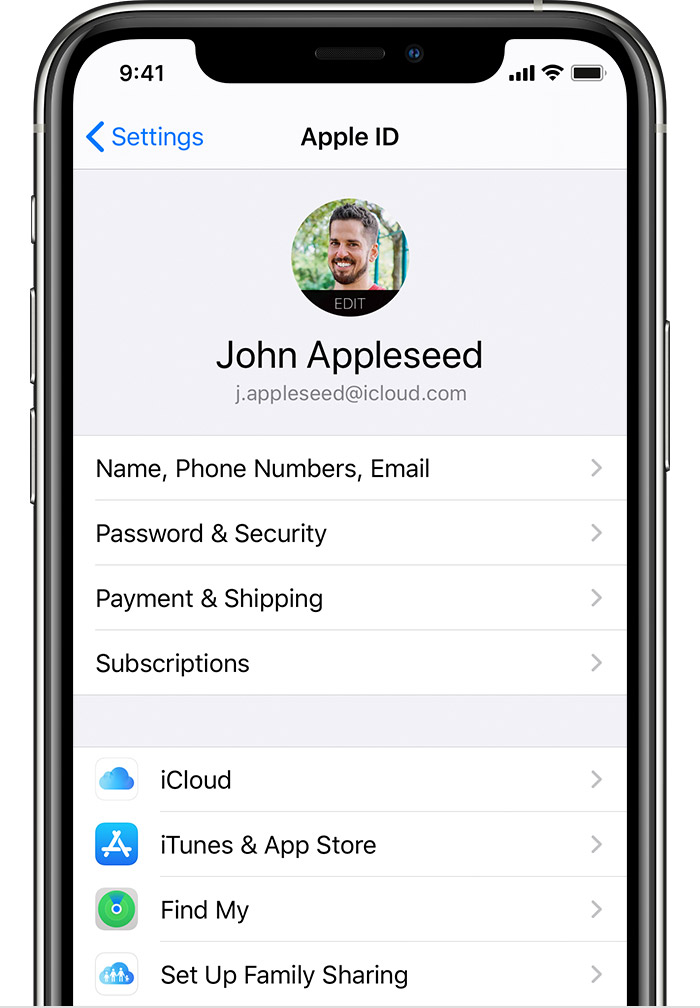The image depicts a silvery iPhone displaying the Apple ID settings page. 

In the upper left corner of the screen, "9:41" is shown, while the upper right corner displays the Wi-Fi symbol, battery level, and signal bars. The page itself is titled "Settings" in blue on the left side, with "Apple ID" prominently in black in the center. Underneath this title is a gray rectangular box containing a circular profile picture of a smiling man with short dark hair and a short dark beard and mustache. He is a white man, and this image is accompanied by a label at the bottom that reads "Edit."

The text "John Appleseed" appears below the photo, followed by "jappleseed@icloud.com." The settings options are listed against a white background with black text: 
1. Name, Phone Numbers, Email 
2. Password & Security 
3. Payment & Shipping 
4. Subscriptions

Below these, there is a gray shaded area followed by additional settings:
- "iCloud," accompanied by a cloud icon
- "iTunes & App Store," with a blue square icon featuring a white "A"
- "Find My," displayed with a green circle icon with a small blue patch
- "Set Up Family Sharing," indicated by a blue cloud icon with a white silhouette of a family holding hands